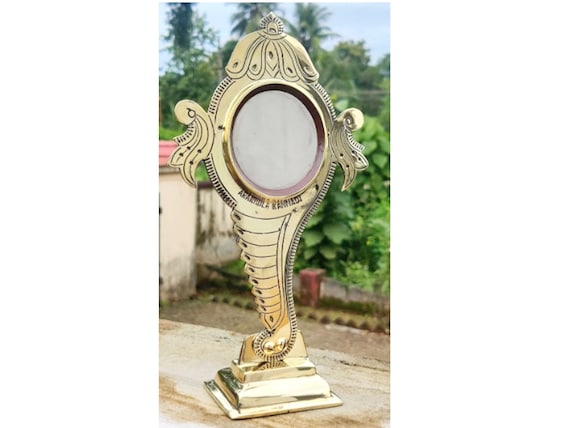The photograph displays an ornate golden monstrance, positioned on a yellowish-brown wooden surface that might be a windowsill or a deck. The monstrance features a circular center, possibly a mirror or host, framed by intricate ornamental designs that evoke imagery from a fairy tale or Disney movie. The base of the monstrance resembles a snake or dragon, contributing to its elaborate appearance. In the background, lush greenery is evident with various trees, including what seem to be weeping willows and larger tree trunks. A red-roofed yellowish-brown building is visible in the left-hand side of the image, along with a strip of blue sky at the top, while vines grow along a fence or wall to the right. The outdoor setting combines natural elements with the mystical, crafted appeal of the monstrance, creating a striking and detailed scene.